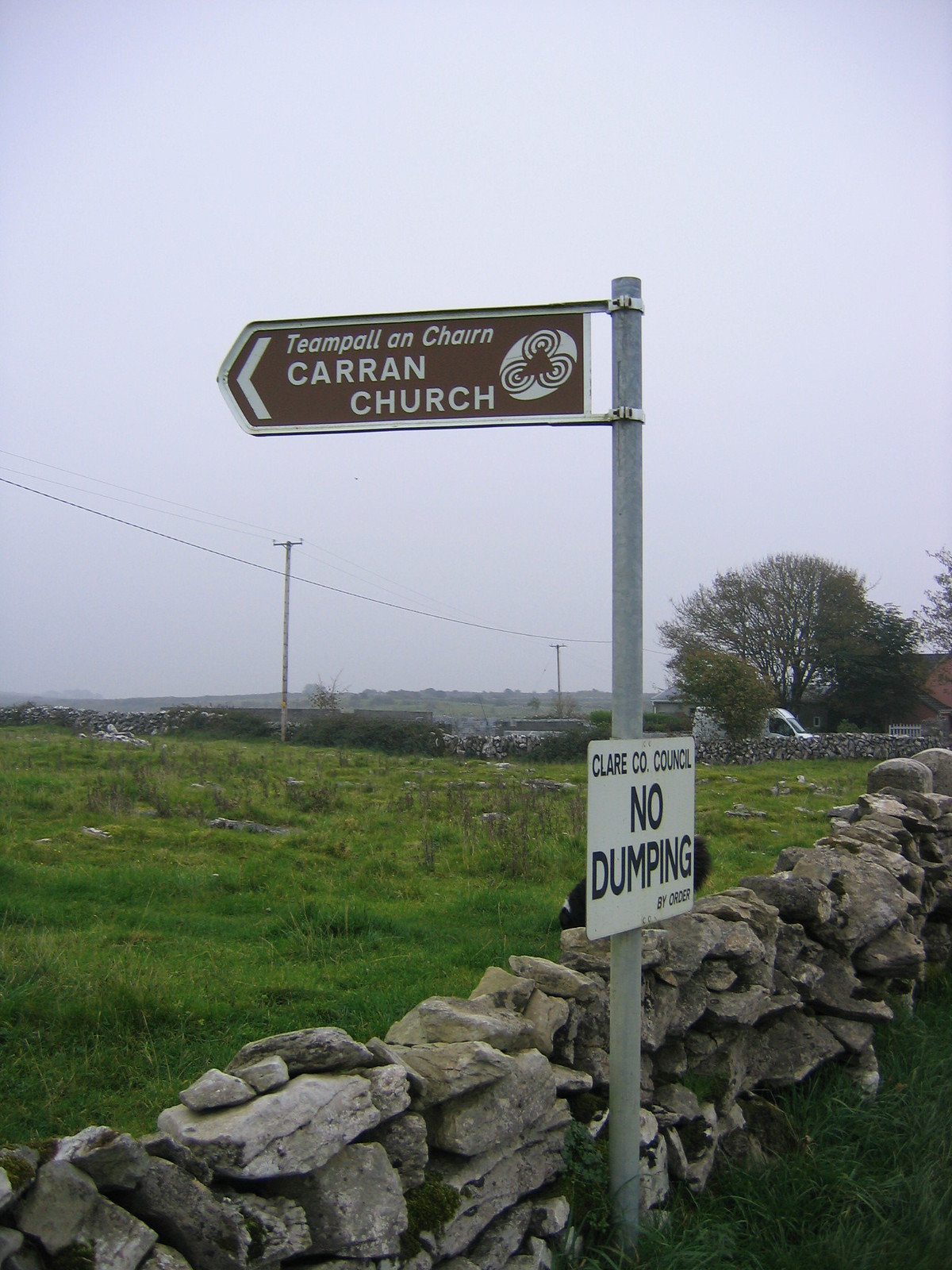In the foreground of the image, a roughly constructed stone retaining wall composed of variously sized and shaped rectangular rocks, including gray, brown, and white stones, extends diagonally from the bottom left corner towards the middle right side, disappearing out of the frame. Moss can be seen growing on one of the stones, adding a touch of green. Above the wall, there is a gray metal pole, approximately 10 to 15 feet tall. Mounted on this pole is a brown sign with white lettering that reads "Carran Church," accompanied by a white arrow pointing to the left. Additionally, a smaller white sign affixed to the pole states "No Dumping" in clear, dark letters. The background features a field with expanses of grass, intersected by two phone lines and dotted with phone towers and a large tree.